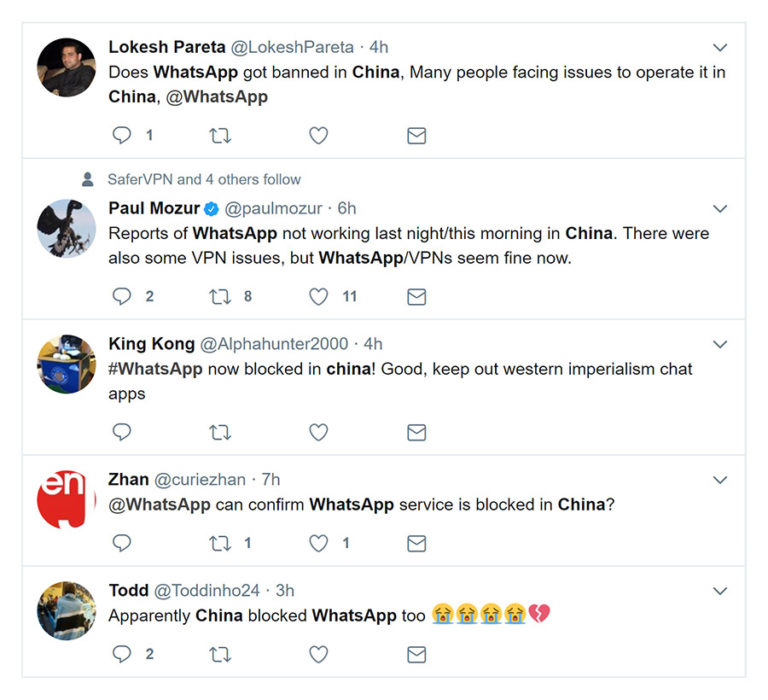This image contains five distinct tweets, organized vertically with a consistent light gray border surrounding the entire layout and separating each individual tweet.

1. **Tweet One**: 
   - On the left side is a profile picture of a man with dark hair, wearing a green shirt, seated on a brown couch.
   - To the right, the username is displayed in bold black text, accompanied by a gray handle.
   - A blue check mark indicates a verified account.
   - The tweet was posted six hours ago and discusses China and WhatsApp over two lines.
   - Engagement metrics show two replies, eight retweets, and eleven likes.
   - Below the text, symbols for comments, retweets, and likes are visible, along with an email-like icon.

2. **Tweet Two**: 
   - The profile picture features a hawk with a brown back, white tail, and brown tip, perched on a branch.
   - The username is presented above this image, also featuring a blue checkmark.
   - This tweet consists of a single line about WhatsApp and China.
   - Engagement: two replies, eight retweets, eleven likes.

3. **Tweet Three**: 
   - Displays the profile picture of King Kong in a blue box.
   - Contains a single line of text followed by one word related to WhatsApp and China.
   - Noted for having no likes, retweets, or replies.

4. **Tweet Four**: 
   - Features a red circular profile picture with white letters "EN" at the top and a "J" down the right side.
   - The tweet has one retweet and one like.

5. **Tweet Five**: 
   - Has a blurry profile picture showing a group of people from behind, some wearing multi-colored hoodies (blue, white, black).
   - The tweet includes one line of text with four crying face emojis and one pink broken heart emoji.
   - Engagement shows two comments.

Each tweet is meticulously arranged to provide clear visual and textual information about the ongoing public discourse around China and WhatsApp.